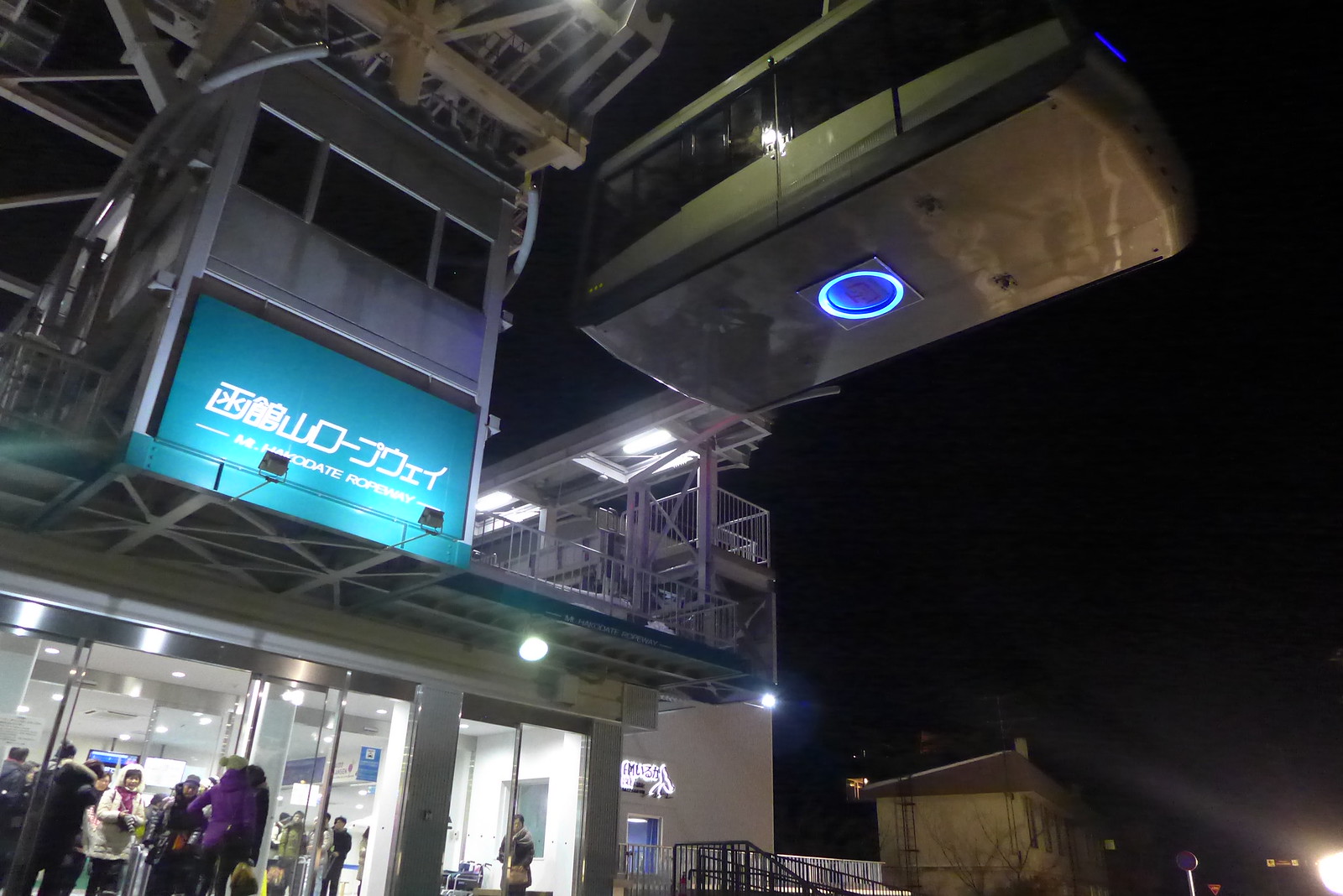In the image, a teal-colored, rectangular sign adorned with white characters in a foreign language—presumably Asian—is prominently displayed on the front of a building. The sign is illuminated by spotlights, although a glare partially obscures some of the text. Above the sign, suspended from a rafter, is a large, square object featuring an illuminated blue circle, light blue on the outer ring and dark blue in the center.

The building's front is primarily glass, with sliding doors framed in stainless steel at the entrance. Numerous people, some with luggage and coats, are gathered around the entrance area, indicating a busy, possibly commercial location. A notable figure is a woman in a white jacket with a pink scarf standing in the doorway.

To the right side, which is cast in darkness, suggesting it's nighttime, there’s a yellow light shining on the bottom right corner. The bottom center of the image reveals a wheelchair ramp with barriers leading up to the building, which adds to the accessible design of the structure.

Overhead, a motorized tram or gondola, resembling a large rectangular box approximately the size of a car, hangs from wires connected to a control tower above the building. This tram appears to be part of a mountainous ropeway system, implied by a partially visible sign that reads "M *something* Date Ropeway," illuminated by a spotlight. Additional buildings, lights, and street poles are visible in the distant backdrop, further suggesting an outdoor nighttime setting. The overall scene is bustling with activity, likely at a ropeway station where people gather to embark on their excursions.